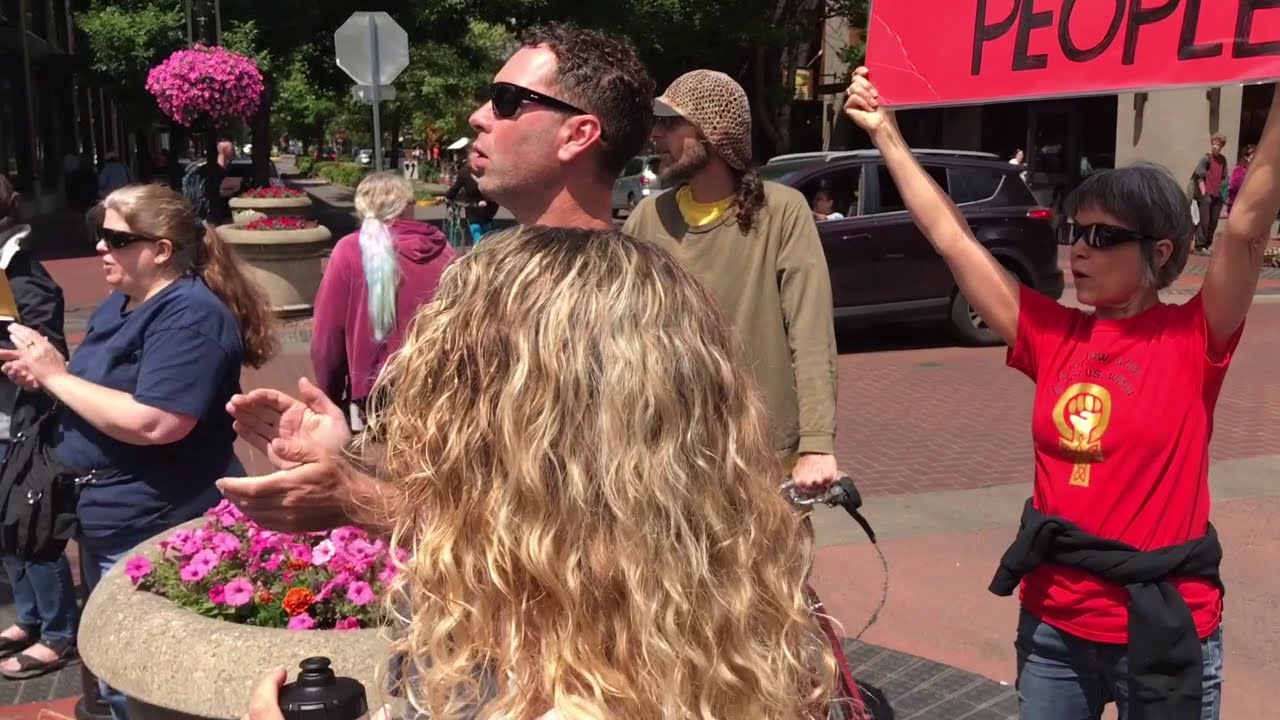The photograph captures a lively outdoor protest scene, possibly in a city or a town's common area, with cars visible in the background. Dominating the right side of the image, a woman sporting short gray hair and sunglasses stands out, wearing a red shirt adorned with a golden fist around a female gender symbol. She has a black jacket tied around her waist, paired with blue jeans, and is holding up a red sign, partially visible, that reads "people" in black letters. The crowd, comprising several individuals, appears engaged and focused, all looking to the left with their hands clapping as if responding to a speaker. Among them is a man in sunglasses and a beige sweater with a knit cap, exuding a hippie vibe, along with women with blonde hair, one of whom has a ponytail. The sunny setting enhances the beauty of the scene, featuring gardens and large stone bowls filled with vivid pink plants, suggesting it might be in a picturesque place like Berkeley.